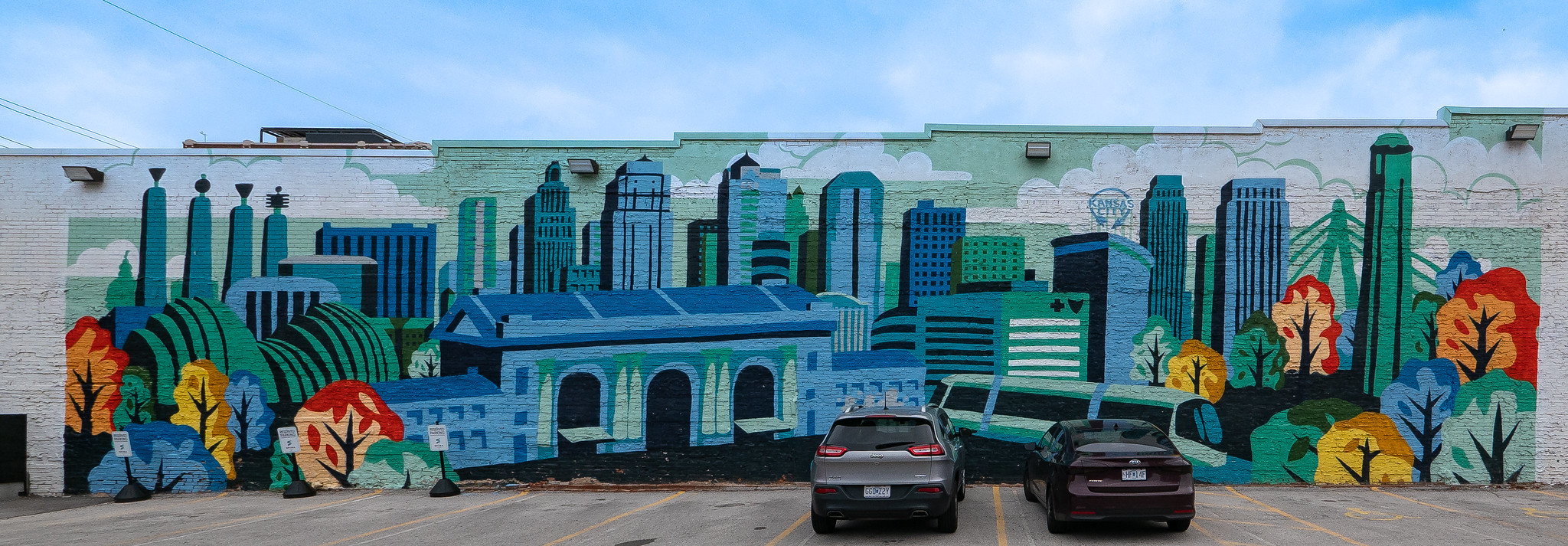The image showcases an intricately painted mural on the side of a brick or cinder block building, which stretches horizontally across the entire frame. The artwork is a vibrant cityscape featuring a cluster of buildings in shades of blue, gray, and green. Prominent in the mural is a building slightly left of center, angled diagonally, featuring three black archways and a roof adorned with blue and lighter blue outlines. Surrounding this structure are various colorful trees, displaying a rich palette of red, yellow, orange, blue, and green, suggesting an autumn scene.

Foregrounded on both sides are detailed depictions of street scenes, including a visible city bus, several parked cars, and even signs indicating reserved parking spots. Above the buildings, the sky is painted in a clear blue with softer, semi-transparent clouds and power lines adding to the urban aesthetic. The mural combines elements of realism with artistic flair, creating a dynamic and picturesque representation of city life.